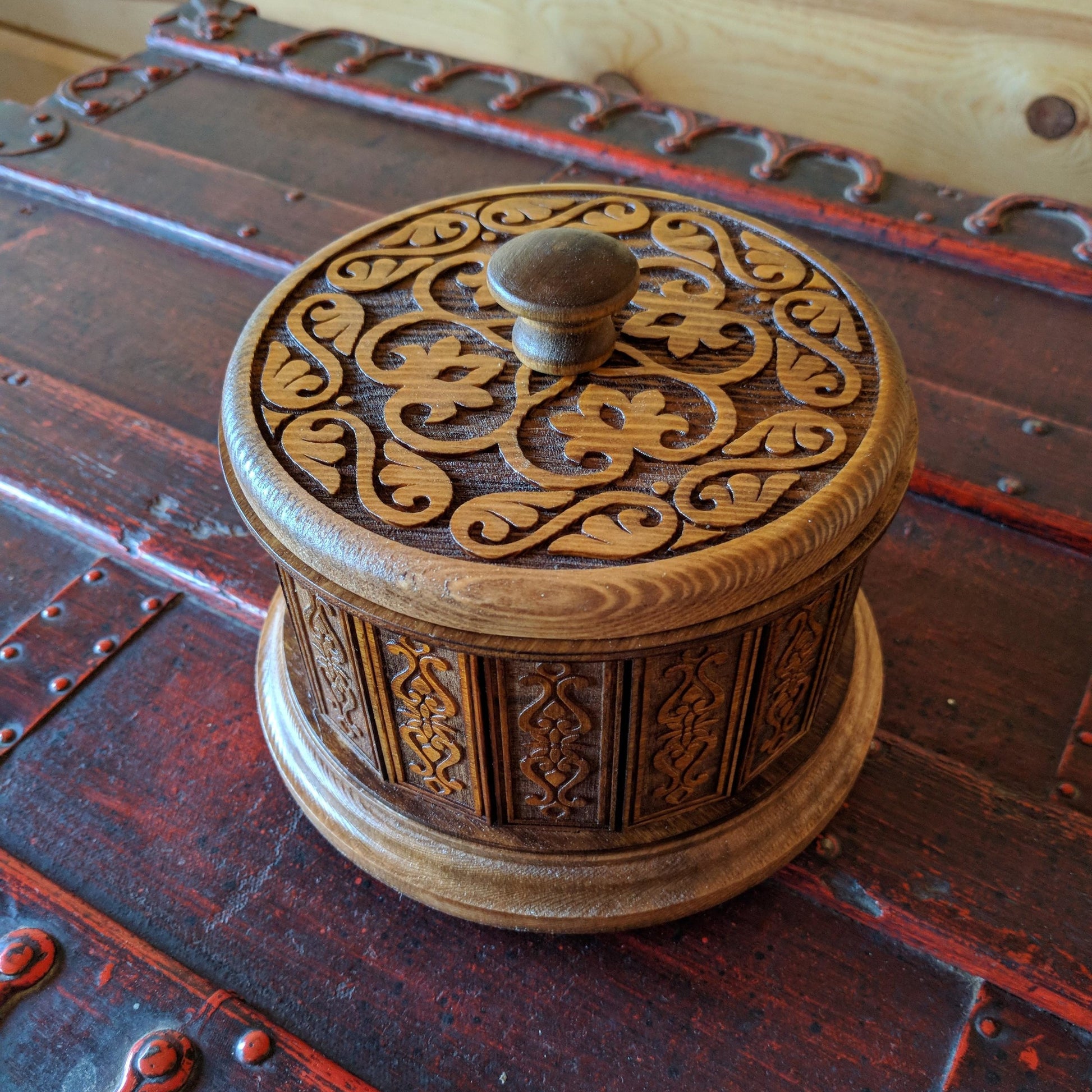The photograph showcases an intricately carved wooden container, cylindrical in shape, prominently placed at the center. The container, stained in a medium dark brown, features repeating floral patterns along its sides and lid, with a simple dark wooden knob for opening. This ornate piece rests atop what appears to be an antique trunk, characterized by its reddish-orange and brown hues, possibly constructed from wood with metal trimming. The background reveals a plain wooden wall with a natural texture, accentuating the vintage and rustic aesthetic of the scene. The image is tightly framed, focusing primarily on the detailed craftsmanship of the wooden container and the antique trunk it sits upon.